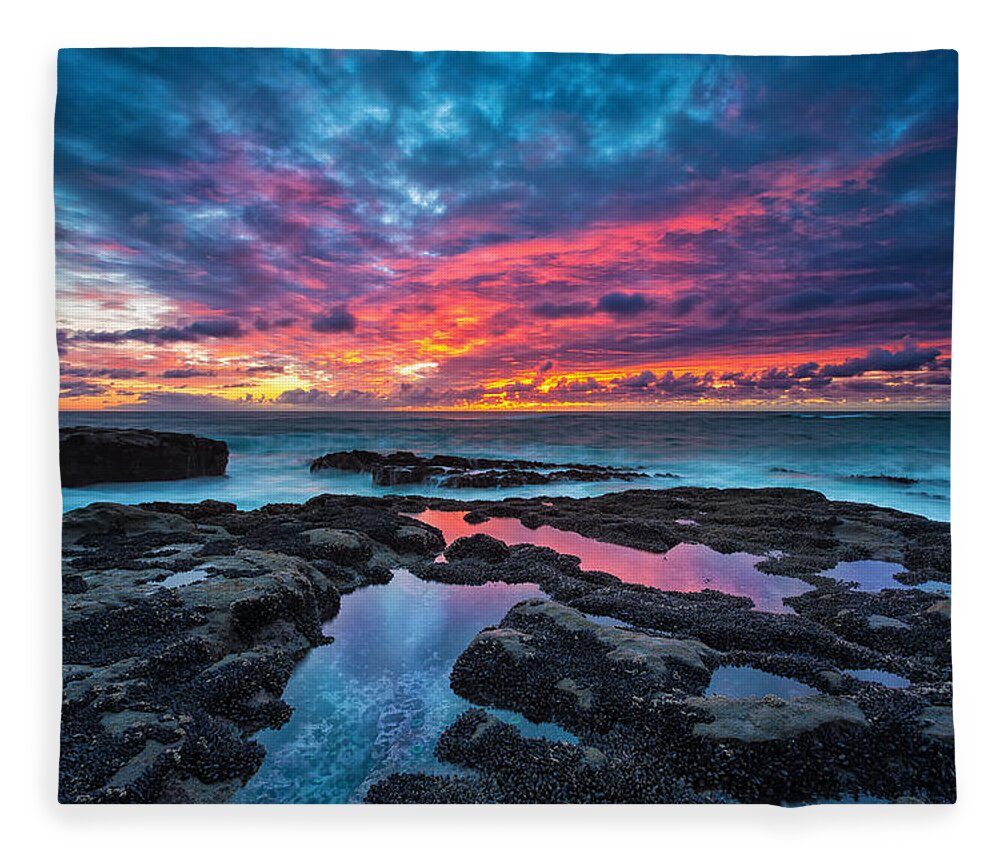This vibrant wall hanging features an exquisite seascape captured in a photograph, meticulously printed on a large square piece of fabric. The scene is depicted from the vantage point of the shore, gazing out towards the expansive sea. In the shallow waters, dark grey rocks offer a stark yet beautiful contrast to the surrounding calmness. The mesmerizing sunset, a symphony of yellow, pink, purple, and blue hues, graces the sky, with the colors artfully diffused amongst the clouds. The same breathtaking hues of the sunset are mirrored on the surface of the sea, creating a harmonious blend of nature’s beauty that invites viewers to lose themselves in its tranquil splendor.